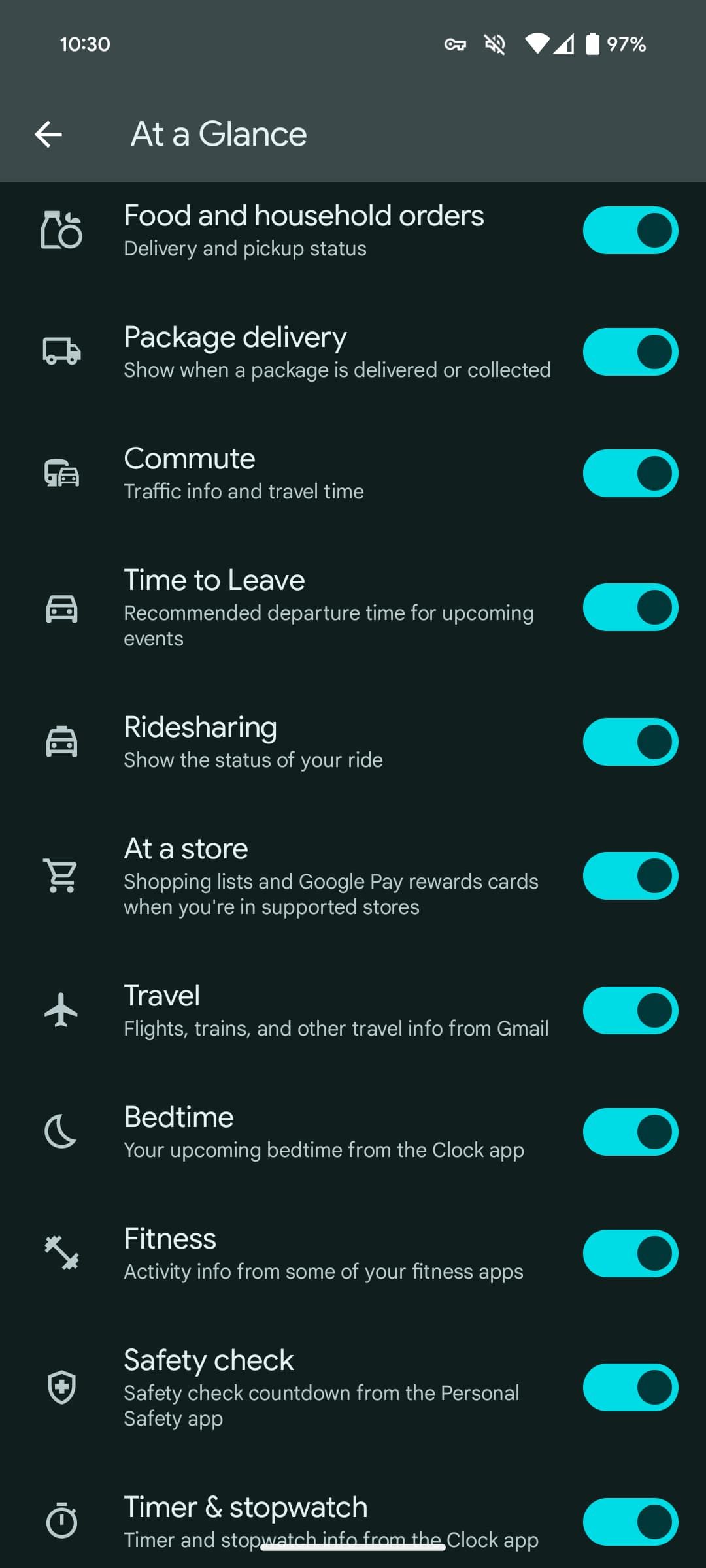This image is a detailed screenshot from a tablet or smartphone interface, presented in a clean and structured layout. The device is set to military time, displaying "10:30" at the top with no AM or PM indicator. Various status icons are also visible at the top: a key symbol, a muted sound indicator, a full Wi-Fi symbol, an almost full cellphone signal, and a nearly full battery at 97%.

Dominating the interface, a bold white arrow pointing to the left is prominently placed adjacent to a section titled "At a Glance" in the center. On the right side of the screen, multiple sliders, all turned on, are displayed with a cyan blue background and black circles, each accompanied by white text for clarity.

Below the "At a Glance" section, various notifications and settings are listed with distinct icons and labels:
1. **Food and Household Orders**: Depicted with a milk bottle and an apple/orange icon, this section in bold white text mentions "Food and household orders", and below it in gray text, "Delivery and pickup status."
2. **Package Delivery**: Illustrated by a truck icon, this section in bold white text notes, "Package delivery," and in gray text, "Show when a package is delivered or collected."
3. **Commute**: Shown with a bus and car icon, the bold white text reads, "Commute" with gray text below, "Traffic and travel time."
4. **Time to Leave**: Represented by a single car icon, the bold white text states, "Time to leave," followed by the gray text, "Recommended departure time for upcoming events."
5. **Ride Sharing**: An icon of a taxi with a small box on top denotes this section, with bold white text saying, "Ride sharing," and gray text, "Show the status of your ride."
6. **At a Store**: A shopping cart icon signifies this section, where the bold white text mentions, "At a store," and gray text, "Shopping list and Google Pay rewards cards when you're in supported stores."
7. **Travel**: Illustrated with an airplane icon, the bold white text reads, "Travel," and the gray text mentions, "Flights, trains, and other travel info from Gmail."
8. **Bedtime**: A crescent moon icon marks this section, with bold white text, "Bedtime," and gray text, "Your upcoming bedtime from the clock app."
9. **Fitness**: Represented by a barbell icon, the bold white text says, "Fitness," and gray text, "Activity info from some of your fitness apps."
10. **Safety Check**: A shield with a cross icon signifies this safety feature, mentioning in bold white text, "Safety check," and gray text, "Safety check countdown from the personal safety app."
11. **Timer and Stopwatch**: A stopwatch icon for this section with bold white text, "Timer and stopwatch," and gray text, "Timer and stopwatch info from the clock app."

Finally, at the bottom, the screen is partially obscured by an oval white bezel, indicating a navigation area.